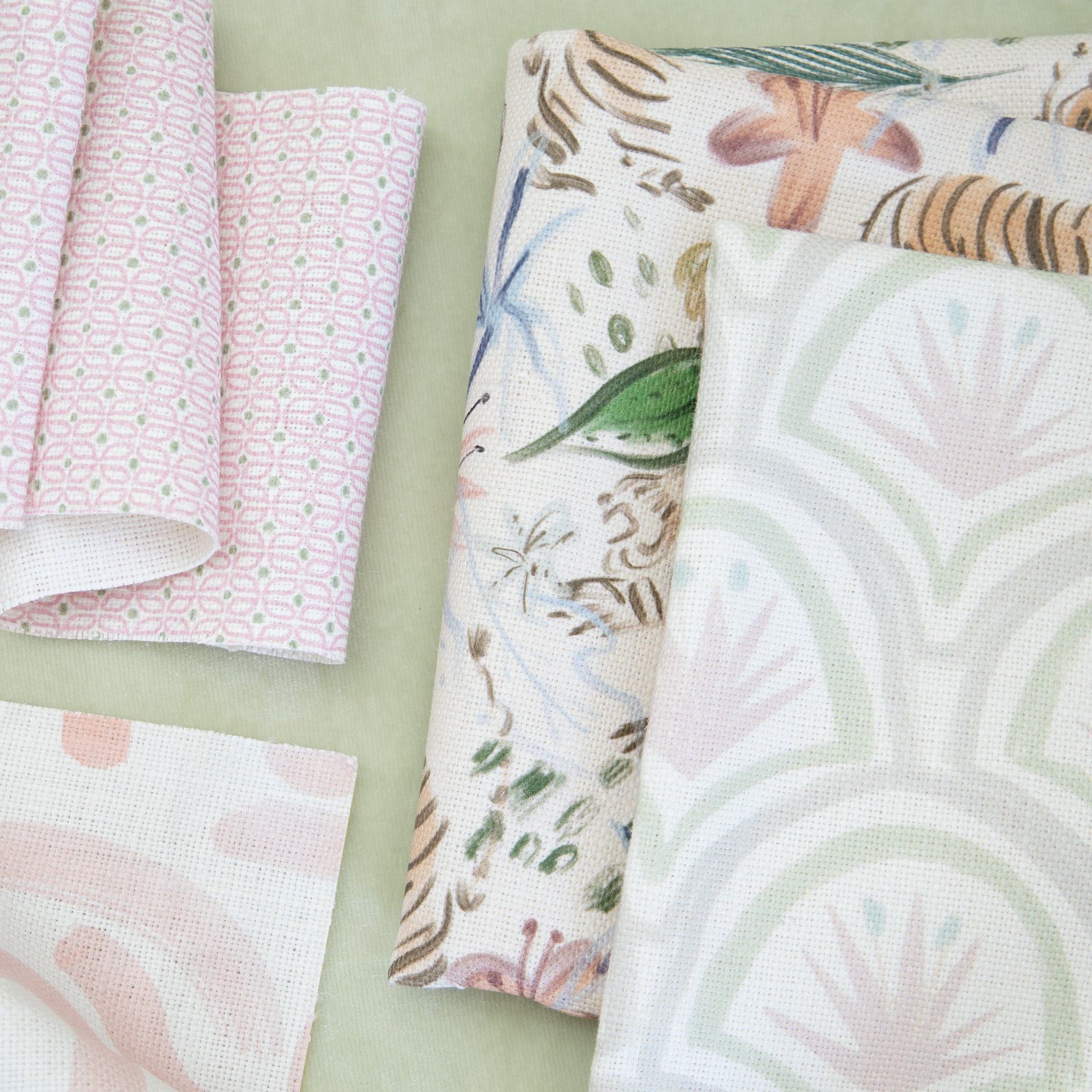The image depicts a stack of five fabrics, with four patterned linens resting atop a fifth base fabric in a minty sea-foam green canvas texture. The top-left fabric features a pink and green pattern of circular motifs with crosses and central blue dots. Below it, on the bottom-left, is a white fabric adorned with subtle, swirly pink brushstrokes and dots. The top-right fabric showcases colorful butterflies, flowers, and mushrooms against a light tan background, while the bottom-right fabric displays a geometric design with a palm leaf silhouette encapsulated in grayscale. Behind the latter is an abstract-patterned fabric, completing a diverse and vibrant collection of textures and designs.